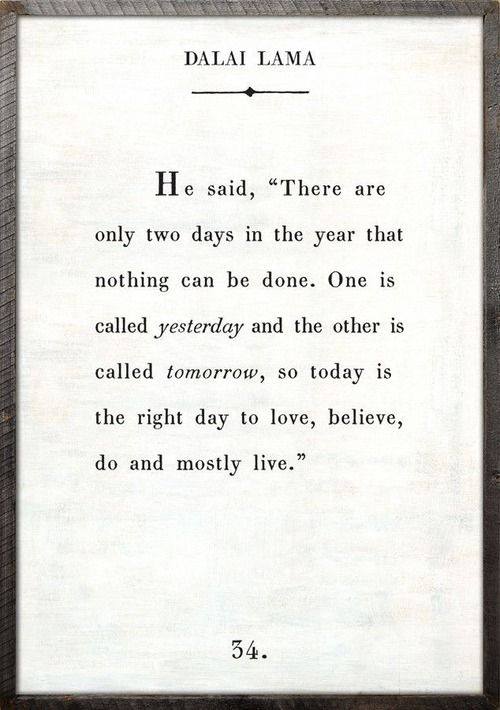The image is a photograph of a framed page from a book. The frame surrounding the page appears to be made of wood, with a grayish hue interspersed with bits of brown, giving it a rustic yet refined look. The page itself has a white background with black text. At the top of the page, it attributes a quote to the Dalai Lama: "He said there are only two days in the year that nothing can be done. One is called yesterday and the other is called tomorrow. So today is the right day to love, believe, and do, do and mostly live." At the bottom right corner of the page, the text "34" is visible, indicating the page number.